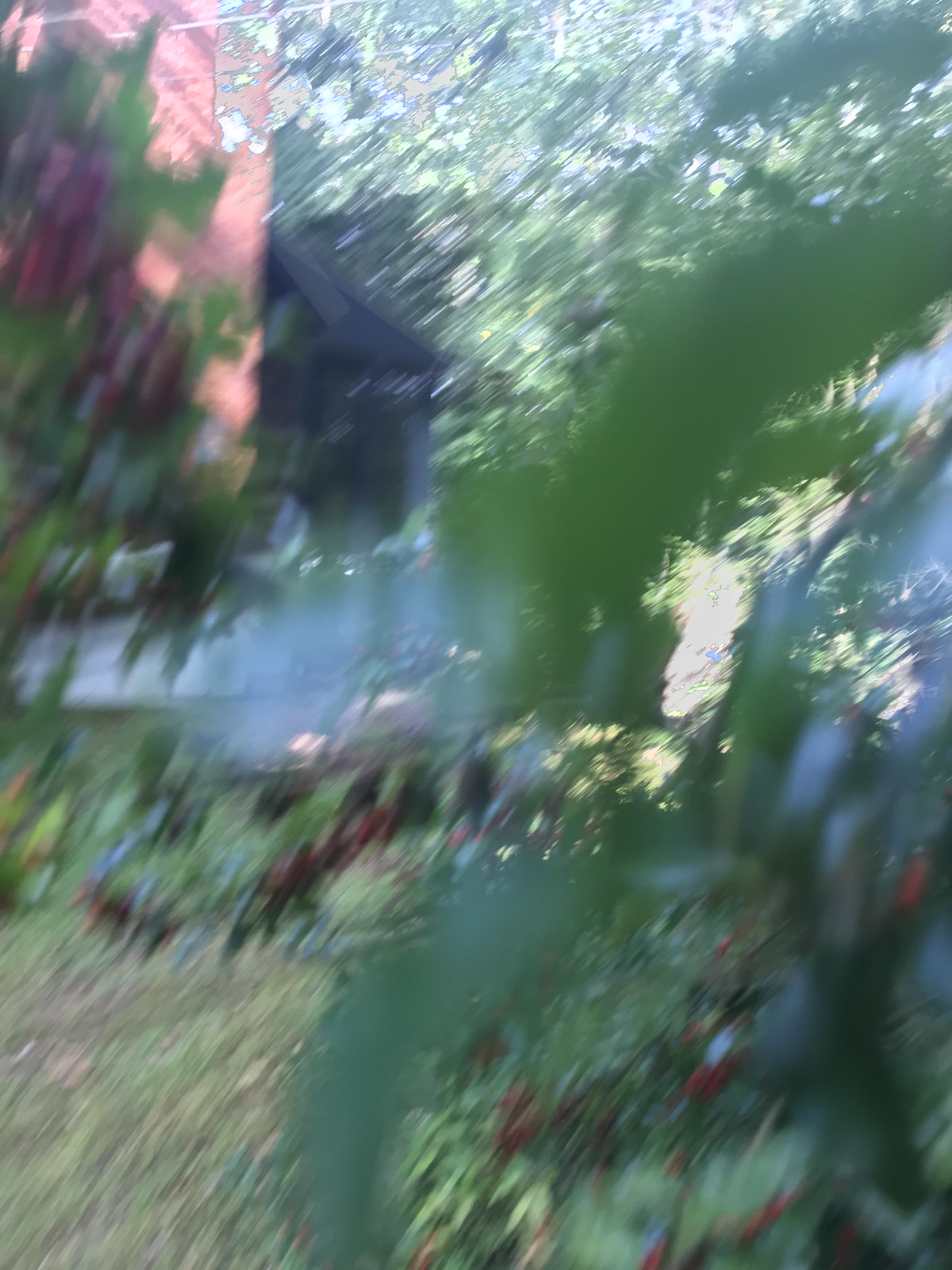Captured from a hidden vantage point amidst dense green foliage, this photo offers a peek into a serene backyard. The photograph appears to be taken from within a bush or tree, emphasizing a sense of seclusion and nature's embrace. Toward the upper left corner, a shadowy structure, likely a dark-colored house, is partially visible, adding an element of mystery against the lush greenery. The scene is framed beautifully by an array of verdant leaves and branches, creating a tranquil and intimate glimpse into someone's outdoor sanctuary.